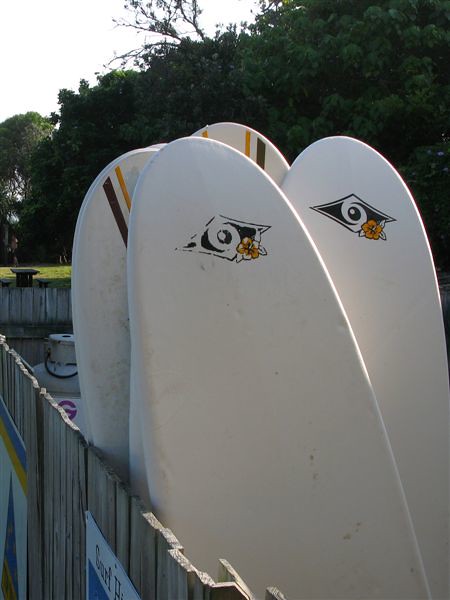This outdoor photograph captures a sunny day scene with a white sky. Central to the image are four white surfboards propped up against a wooden fence, which bends at a 90-degree angle, forming a corner. Two of the surfboards, positioned at the front, feature a distinctive design: an elongated diamond shape with a brown eye in the center and an orange flower near the lower right corner. Behind them, the other two surfboards display vertical stripes, with thick brown lines on the outside and thinner yellow lines on the inside. In the foreground, the lush green grass is bathed in sunlight, while the background showcases dense green bushes and trees. A few signs of varied colors, although not fully legible, are affixed to the fence. Additionally, a propane container is partially visible on the opposite side of the fence. The scene exudes a relaxed and serene atmosphere, emphasizing the detailed interplay between natural elements and human-made objects.